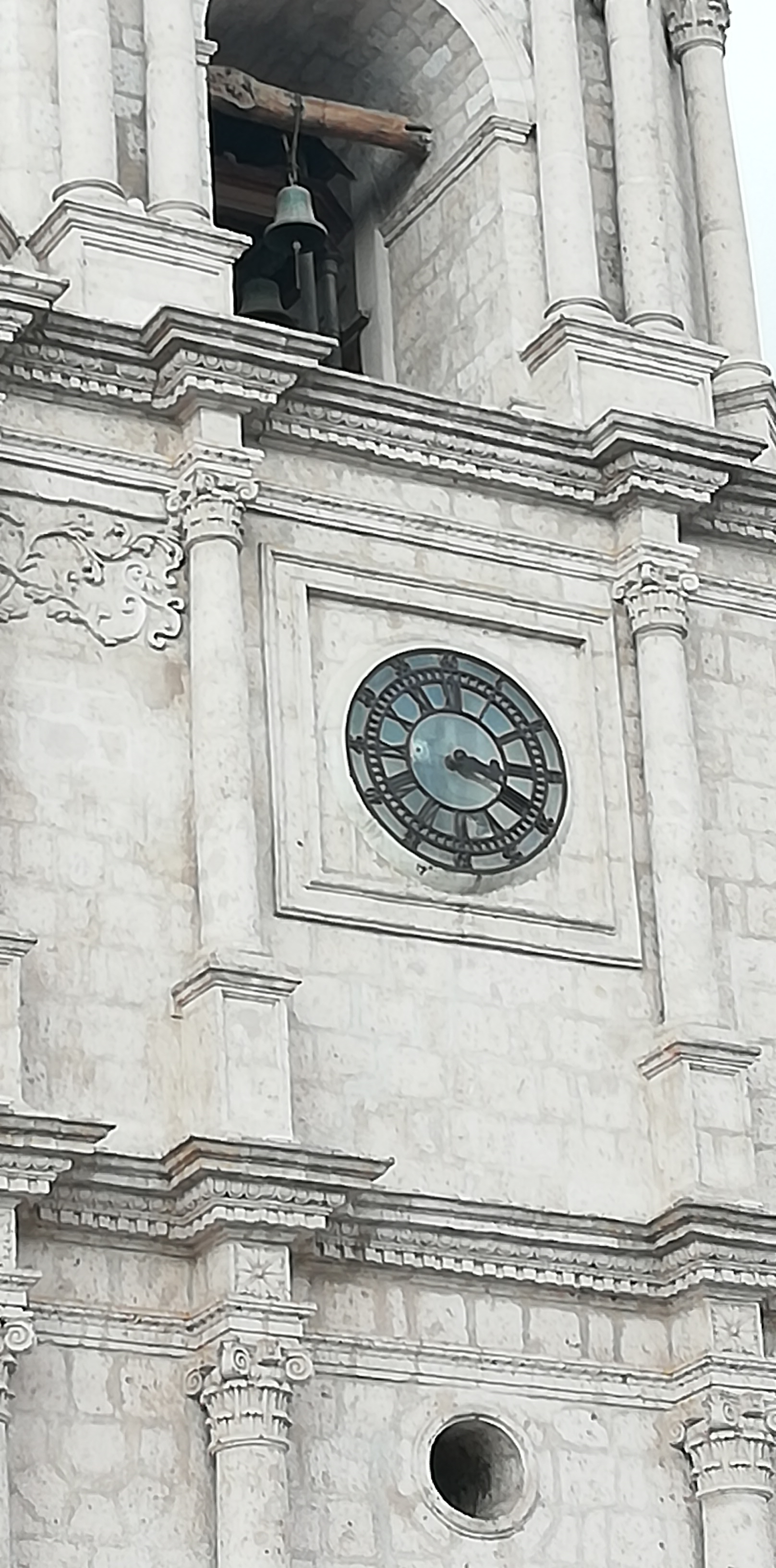The image depicts a historic, light gray bell tower with an intricate architectural design reminiscent of a Roman or classical style. At the very top of the tower is a domed opening housing a dark gray-black bell, suspended from a wooden beam. Directly below the bell, the structure features an ornate band of decorative plinths and columns that span the full height of the building, adorned with carved swirls and elaborate designs. 

On the middle section of the tower’s façade is a large circular clock with a clear glass face, displaying the time with black hands and Roman numerals. The time appears to be approximately 3:20. Just beneath the clock, there is a circular cut-out in the masonry on the lower section of the wall—possibly intended for drainage or other functional purposes. The church-style building exhibits significant historical character through its detailed carvings and structured elegance.